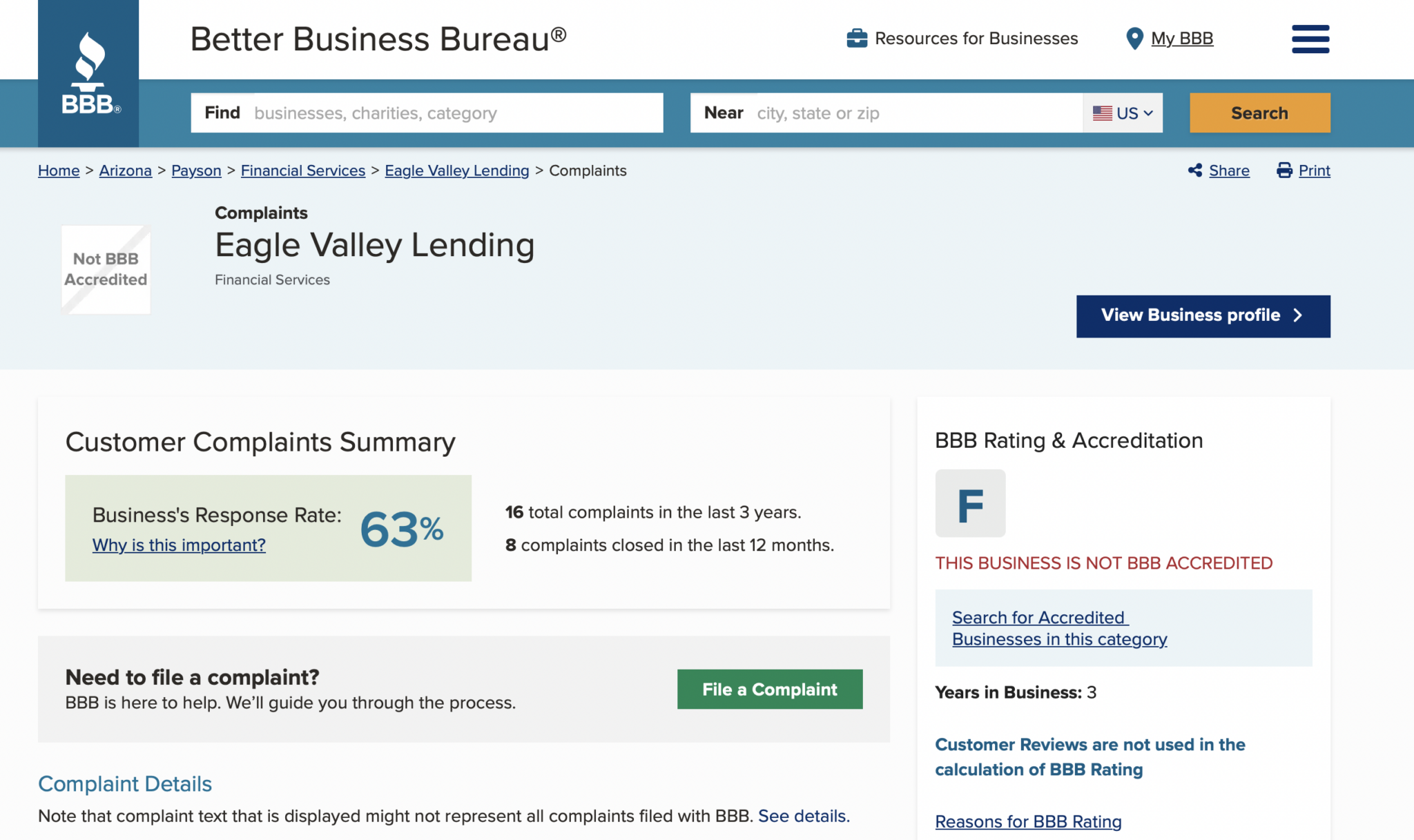This image, sourced from the Better Business Bureau (BBB) website, prominently features the BBB's iconic logo on the left—a white flame set against a navy blue rectangle with the letters "BBB" prominently displayed. Adjacent to this logo, there are two search fields: one labeled "Find" for entering the type of service or business you are looking for, and another labeled "Near" where users can input their city, state, or zip code. At the top of the page, there are navigation options allowing users to access resources for businesses or their personal BBB profile under "My BBB." A distinct yellow rectangle labeled "Search" invites users to initiate their query.

As you scroll down, the page introduces a section on complaints, specifically detailing issues related to "Eagle Valley Lending." This segment includes a navy blue rectangle on the right which links to the business profile under "View Business Profile." Below this, a "Customer Complaint Summary" provides key statistics: a business response rate of 63%, 16 total complaints in the last three years, and 8 complaints closed in the last 12 months. Towards the bottom, there is a green button labeled "File a Complaint" for users needing to report an issue.